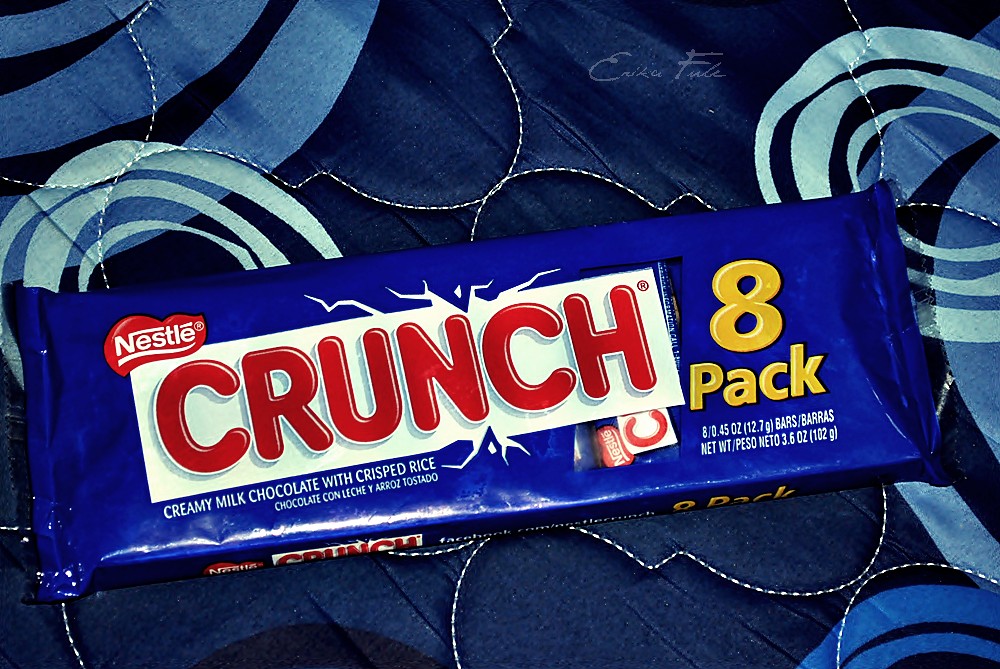This detailed image captures a Nestle Crunch bar package, explicitly marked as an 8-pack of miniature bars. The packaging prominently features the iconic blue background with a large, red "Crunch" logo set within a white rectangular text box across the middle. To the right of the logo, the text "8-pack" is distinctly written in yellow. Above the logo, the word "Nestle" is displayed in white letters, accompanied by their recognizable red heart logo. Below, the package also highlights in white text: "creamy milk chocolate with crisped rice." This rectangular package is laid out on a backdrop that appears to be a blue blanket with intricate designs. The blanket showcases varying shades of blue with light blue swirls, dark blue lines, and white stitching patterns, creating a unified blue theme in the image. Additionally, an artist's cursive signature, reading "Erica F.", subtly appears within the composition.